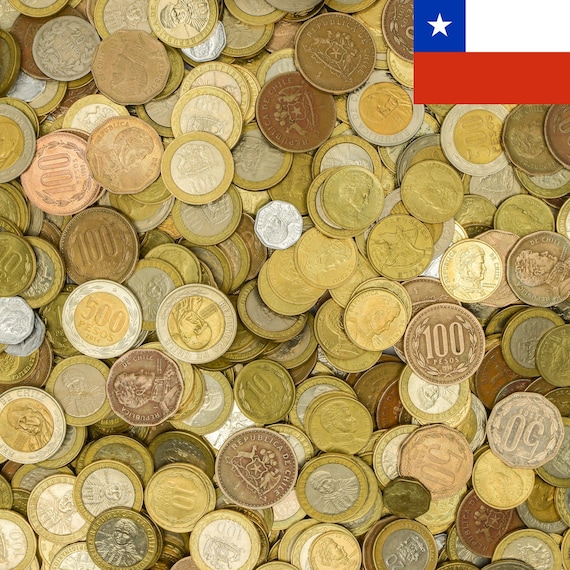This photograph showcases a diverse collection of coins, predominantly featuring Chilean pesos. The coins vary in denominations including 50, 100, and 500 pesos, and the majority are golden, with some bronze and a few smaller silver coins mixed in. Notably, one coin displays the emblem of the Republica de Chile, featuring an eagle and a deer flanking a shield. The coins also exhibit various inscriptions, and several bear the likeness of historical figures. In the top right corner of the image, the flag of Chile—characterized by a blue square with a white star, and red and white bars—adds context to their origin. Among the predominantly Chilean coins, there are a few American pennies likely featuring Abraham Lincoln, suggesting a collection of international currency. The photo captures what appears to be hundreds of coins, highlighting both their differing sizes and intricate details.